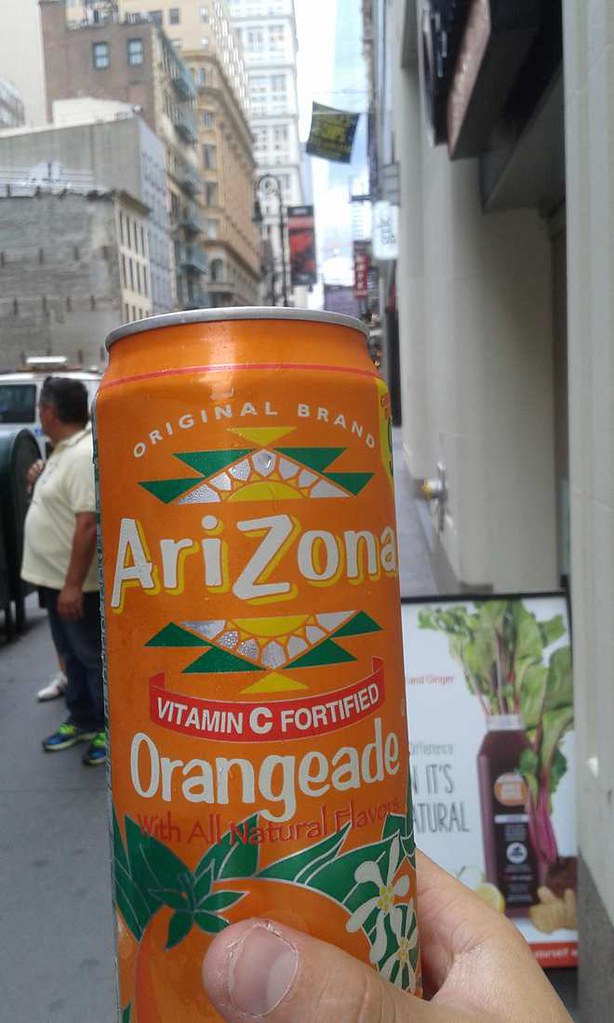In this vibrant urban snapshot, a close-up photograph captures a tall, orange can of Arizona Orangeade held by a Caucasian man with his right hand. The can prominently displays the label "Original Brand Arizona Orangeade, Vitamin C Fortified with All Natural Flavors." To the left of the frame, a man wearing a white short-sleeve shirt looks off to the side, partially obscuring a white van parked behind him. The backdrop reveals a bustling cityscape, with towering buildings of varying colors – a white one, a tan one, a gray and tan structure, and a red brick façade. The scene is bathed in daylight, evident from the sunlight reflecting off the buildings and the clear, blue sky overhead. Additionally, a company sign is subtly visible in the background, adding a touch of commercial life to the image.